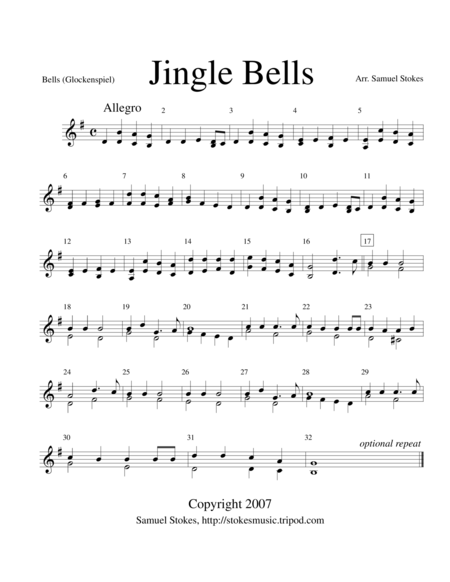The image depicts a printed sheet of music for "Jingle Bells." At the top left corner, in small black text, it reads "bells" followed by "glockenspiel" in parentheses. Centered at the very top in large, bold black letters is the title "Jingle Bells." To the right of the title, it states "Arrangement by Samuel Stokes" in black text. The topmost section on the left side features the term "Allegro" indicating the tempo. The sheet includes numbered measures from 2 to 32 across several lines of musical notation, with music notes distributed across these lines. At the top right corner, the name "Samuel Stokes" appears again. At the bottom of the music lines, the notation indicates an "Optional Repeat." Lastly, at the very bottom center of the page, it says "Copyright 2007 Samuel Stokes" followed by a URL: "http://stokesmusic.tripod.com," all in black text on a white background.